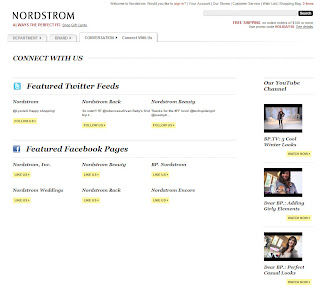This image features a Nordstrom website. At the top, the Nordstrom logo is prominently displayed against a white background. On the left-hand side, there are two major sections in large font. The first section, labeled "Featured Twitter Feeds," showcases three different Twitter feeds: Nordstrom, Nordstrom Rack, and another that appears to be Nordstrom Receiving, although the text isn't fully legible. Below this, the section "Featured Facebook Pages" offers links to six different Facebook pages, each link presented in a yellow box.

On the right-hand side of the page, three videos are listed vertically under the heading "Our YouTube Channel," though the font is too small to read the titles clearly in this image. There is also a search bar located in the upper right-hand corner.